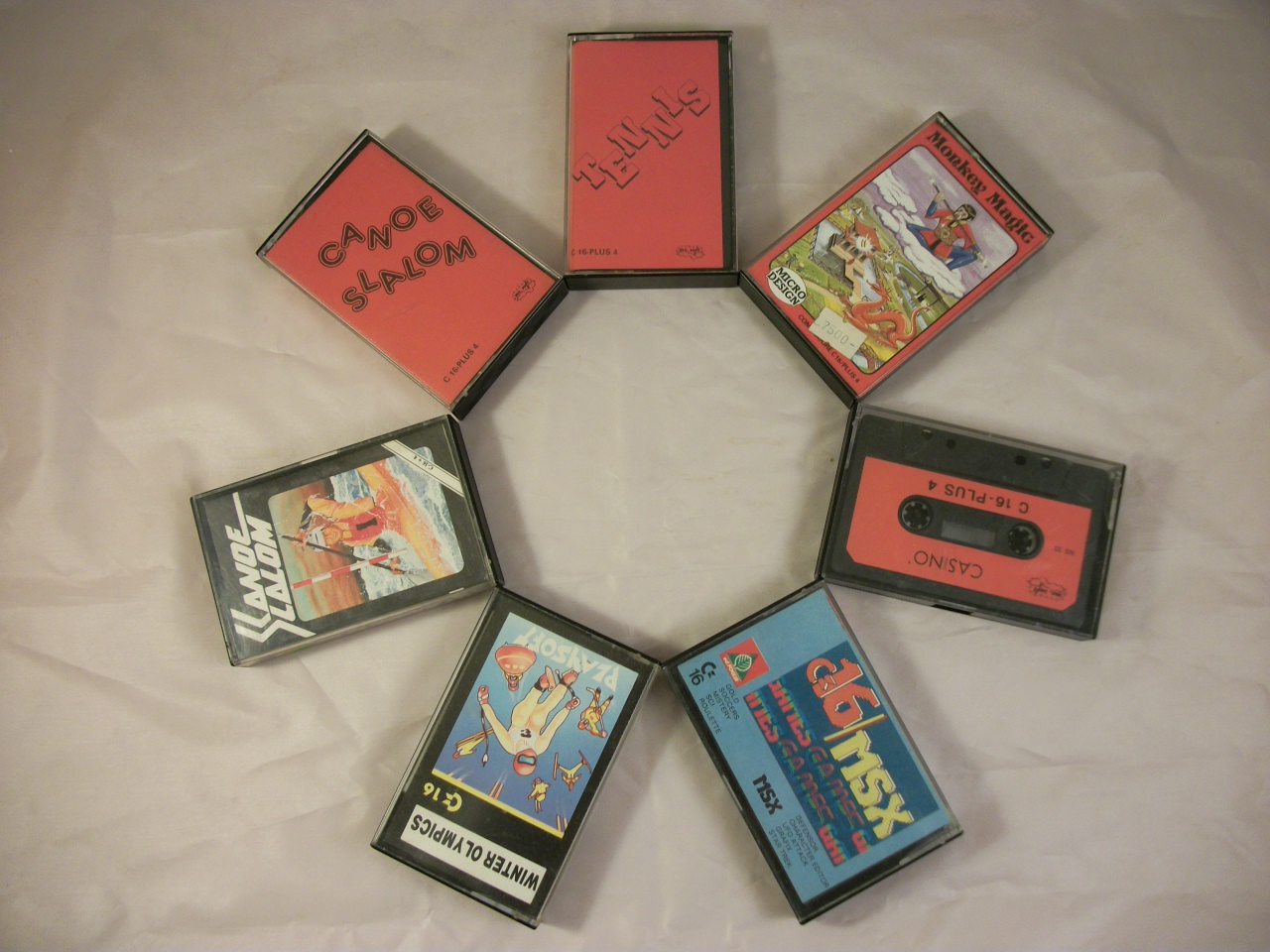The image displays a nostalgic collection of vintage cassette tapes, each encased in its original packaging, arranged in a circular, star-like formation on a cream-colored, wrinkled background, possibly a bedsheet. There are seven cassettes in total, showcasing a variety of colors and designs. On the far right, there is a distinctive tape cassette labeled "Casino C16 Plus 4." Next to it, a case for "Monkey Magic" features an illustration of a monkey amidst clouds. Another red case simply bears the word "Tennis." Positioned at the top left is a red case for "Canoe Slalom," accompanied by a similar black-background case depicting a man in a canoe. At the bottom left, a "Winter Olympics" cassette showcases a skier. Finally, at the bottom right, a light blue package with red and yellow text reads "MSX C16 Games Games Games." The collection demonstrates a blend of vibrant visuals and text, creating a visually interesting and nostalgic snapshot.